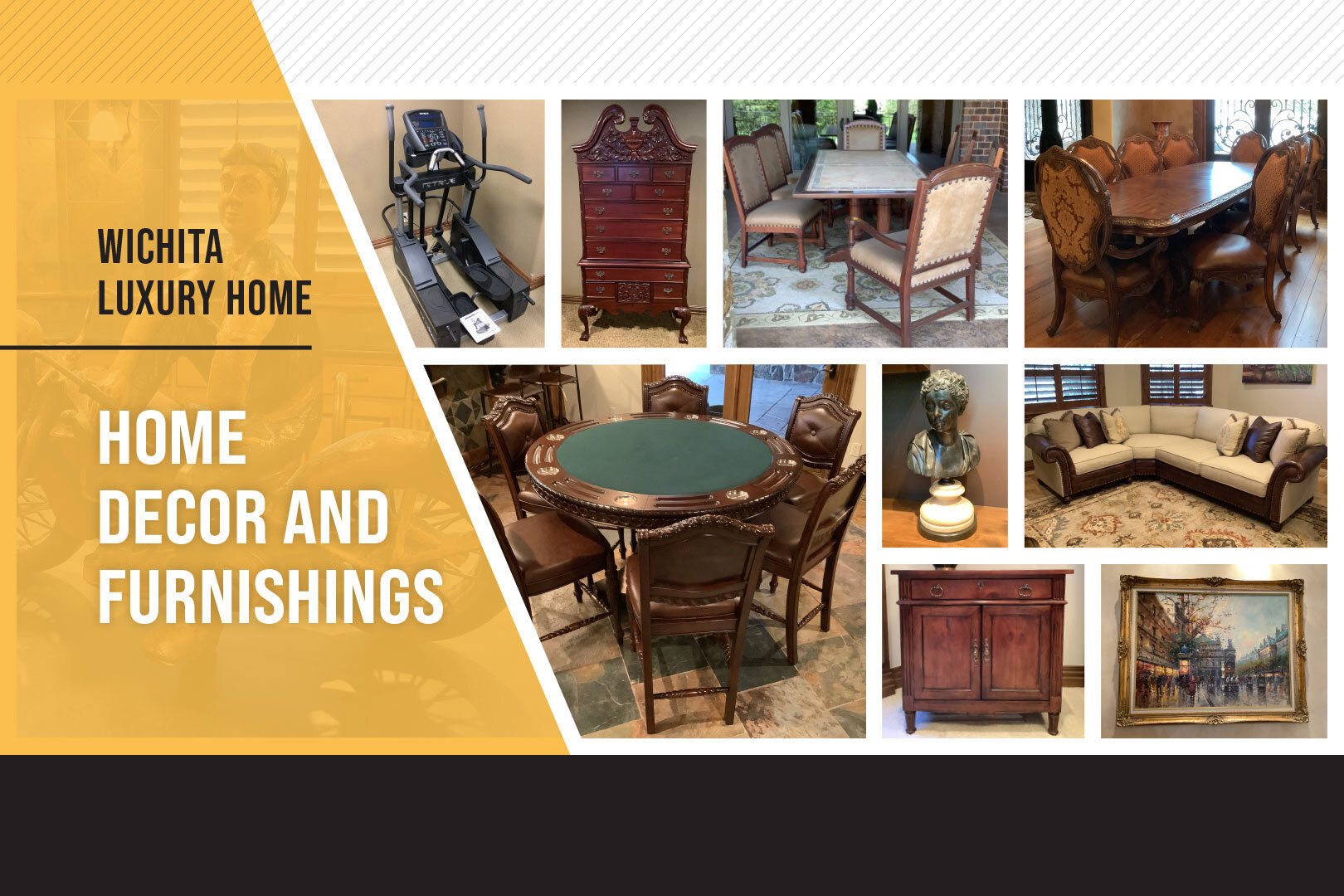This advertisement from Wichita Luxury Home, displayed in a horizontal rectangular frame with a black border at the bottom, showcases an array of home decor and furnishings. On the left side, a reddish-tan polygon features the text "WICHITA LUXURY HOME" in bold, black uppercase letters, and below it, "HOME DECOR AND FURNISHINGS" in white uppercase letters. The remaining right side of the frame is filled with nine photographs displaying various traditional furniture pieces and other home decor items. These include wooden dining sets, an L-shaped sofa with beige upholstery and pillows, a circular poker table surrounded by chairs, several wooden cabinets, a long dining table, a classic-style painting, a bust, and an exercise machine resembling a stairmaster. This advertisement encapsulates the luxurious offerings from Wichita Luxury Home.